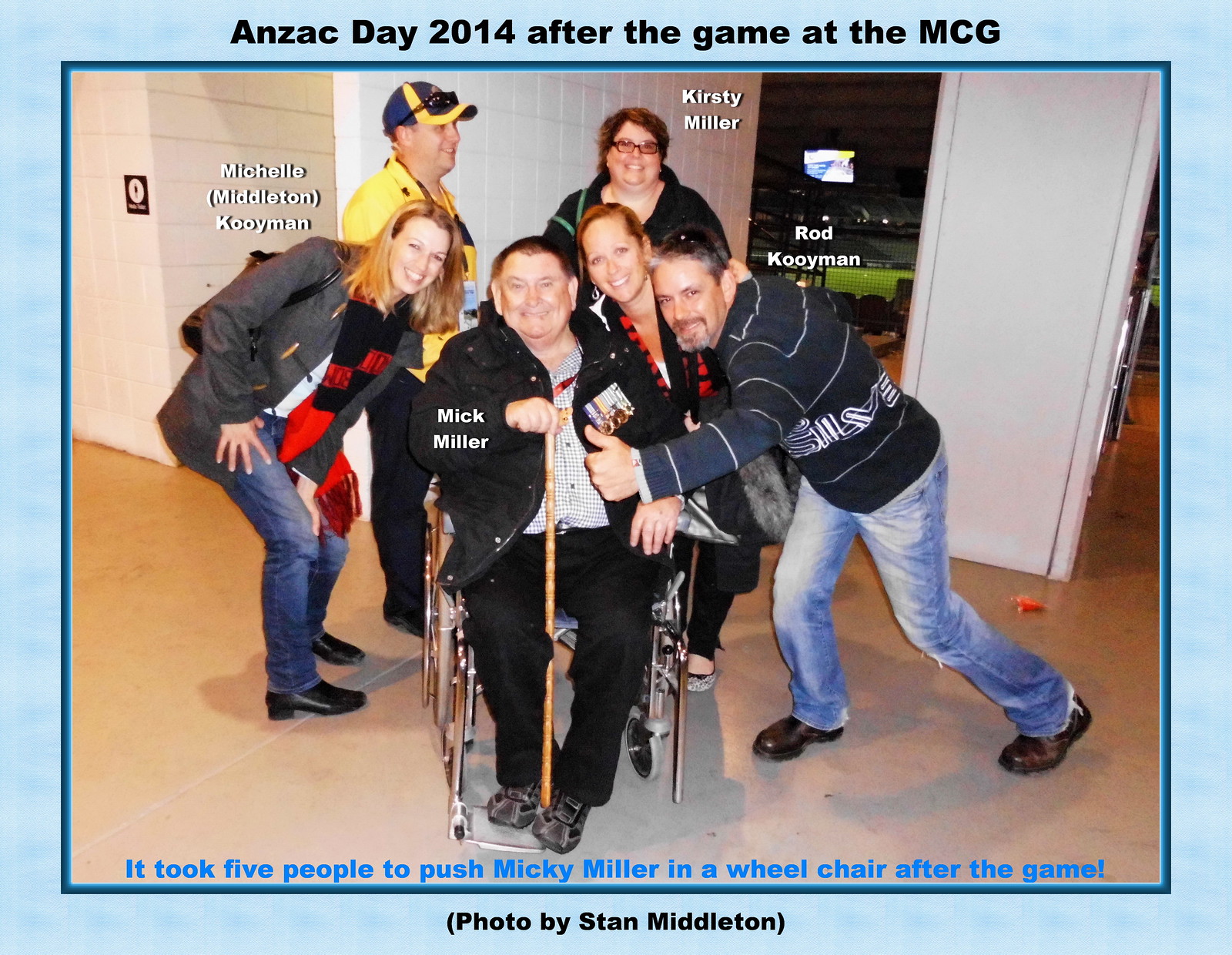The photograph, bordered by a half-inch blue frame, captures a poignant post-game moment on Anzac Day 2014 at the MCG in Australia. At the heart of the image, Mick Miller, seated in a wheelchair and dressed in a black jacket and pants while holding a walking stick, is the focal point. Surrounding him are six individuals. To his left stands Michelle Middleton Cooeyman, identifiable by her blonde hair, gray jacket, blue jeans, and red and black scarf. Behind Michelle is a man wearing a yellow and blue hat with sunglasses perched on top, donned in a yellow shirt and black pants. Slightly further back is Kirstie Miller, sporting glasses, dark hair, and a black jacket. To Mick's immediate right is a red-haired woman in black attire, whose name is not provided. Farther to the right, leaning in with a thumbs up, is Rod Cooeyman, distinguished by his grayish hair, goatee, sunglasses on his head, sweatshirt, and blue jeans. The background faintly reveals a green field and stadium seating, suggesting the scene is set within an arena. The caption at the bottom notes, "Photo by Stan Middleton," emphasizing the communal effort it took—five people—to assist Mick Miller after the game.